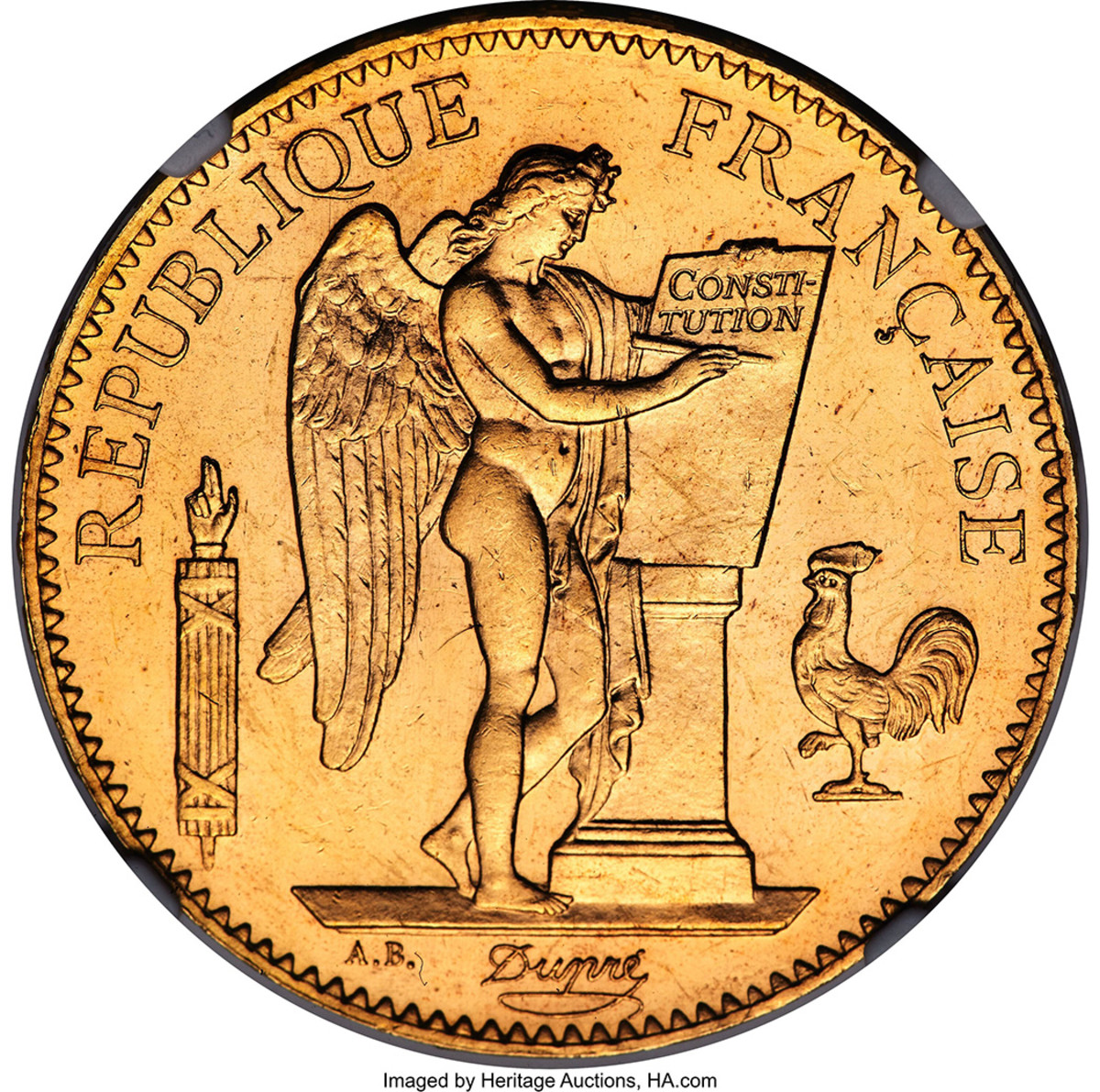This is a detailed photograph of an antique, metallic coin or medallion with a burnished, orangey-brassy hue. The centerpiece features a nude angel with long hair pulled back, wings spread, and a cloth draped over part of the body. The angel, holding a pin in its right hand, appears to be inscribing the word "Constitution" on a large stone pillar. Below the pillar, the name "Dupree," spelled "D-U-P-R-E," is etched, and to the left, the initials "A.B." can be seen. Surrounding the central image, a zigzag pattern adorns the coin's border. On the top, flanking either side of the angel, the inscription "Republique Francaise" signifies its French origin. Additionally, on the right side of the pillar is a rooster with one leg lifted, and on the left, a torch held by a hand making a specific gesture with two fingers extended. Four small tabs, differing in color from the main body, are placed at 10:30, 1:30, 4:00, and 7:00 positions, likely securing the coin to another surface.